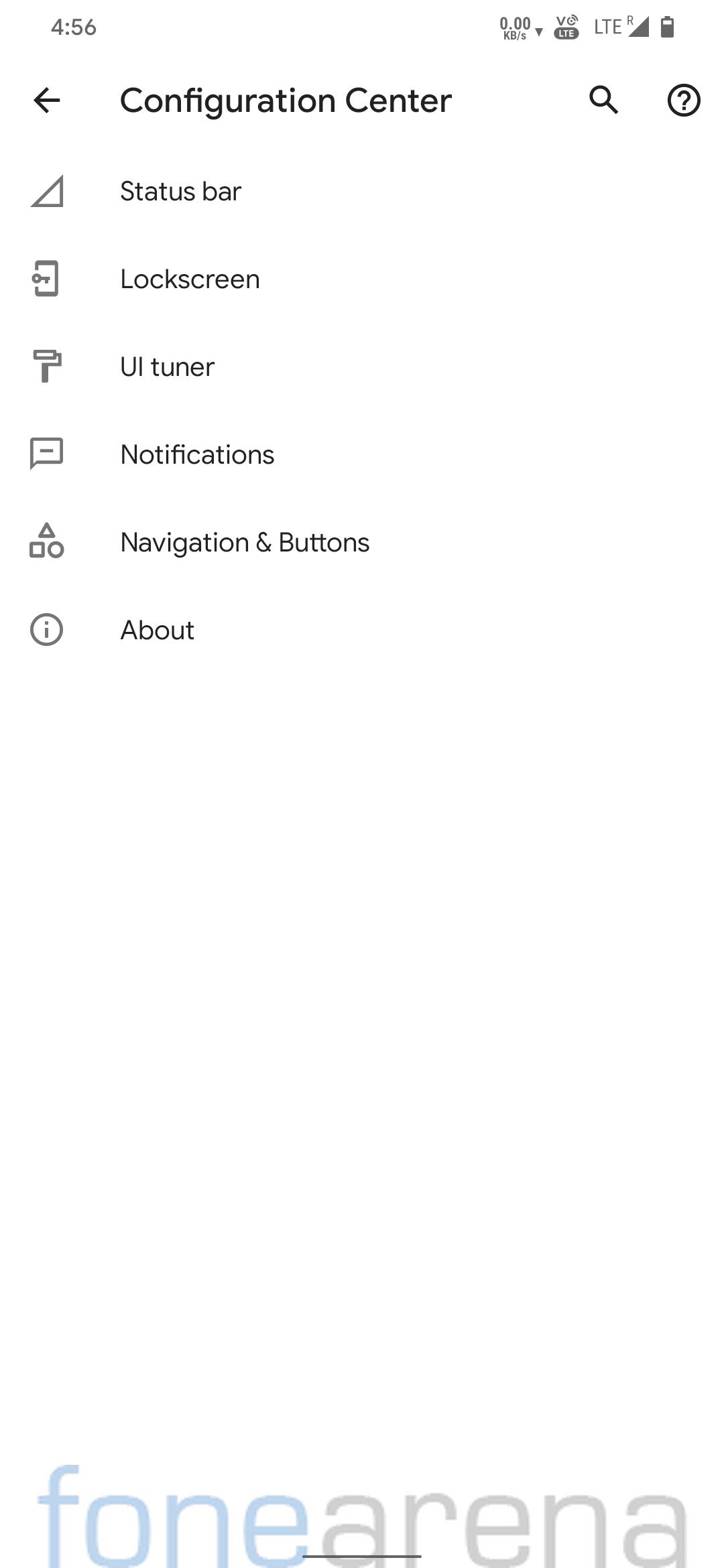The image features a comprehensive view of a Configuration Center interface on a smartphone screen. At the bottom, a watermark reads "Phone Arena," with "Phone" stylized in blue and "Arena" in grey, using the phonetically spelled term "F-O-N-E arena."

The top of the interface displays "Configuration Center" in black text. On the top-left corner, there is a black back button, while the top-right corner houses two black icons: a search icon and a help icon, against a white background. 

Directly below the header, you can see several configuration options. The first option, labeled "Status Bar," is accompanied by a grey network signal icon. The second option, "Lock Screen," features a grey screen lock icon. Following that is the "UI Tuner" option, represented by a grey paintbrush icon.

Continuing down, the "Notification" section includes a grey notification icon. Below that, the "Navigation and Buttons" section displays three grey shapes: a triangle, a square, and a circle. The final section, labeled "About," includes a grey circle icon with an 'i' inside, indicating information.

The clean design and monochromatic icons provide a user-friendly and straightforward configuration interface.